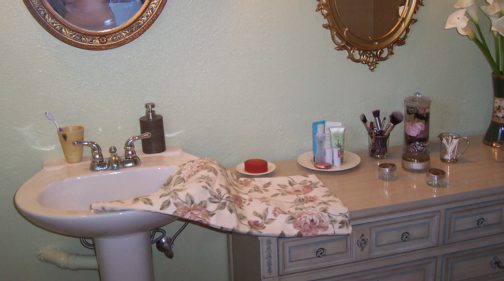This image captures a spacious room that might either be a large bathroom or a bedroom with a sink. The room has a semi-historic European ambiance, reminiscent of older buildings. In the left-hand corner, a classic white porcelain pedestal sink is prominently featured, with visible silver water controls and PVC piping beneath. Adjacent to the sink, there's an ivory white bureau with tan accents, modest in height, resembling a dresser. The wall space above the sink is adorned with an oblong-shaped, gold-framed mirror, positioned centrally. To its right, over the dresser, another gold-framed mirror hangs, this one oval and slightly lower, showcasing intricate design work around its edges. On the far right side of the dresser, a striking black vase with a central gold and cream design holds several white daffodils, adding a touch of nature to the elegant setting.